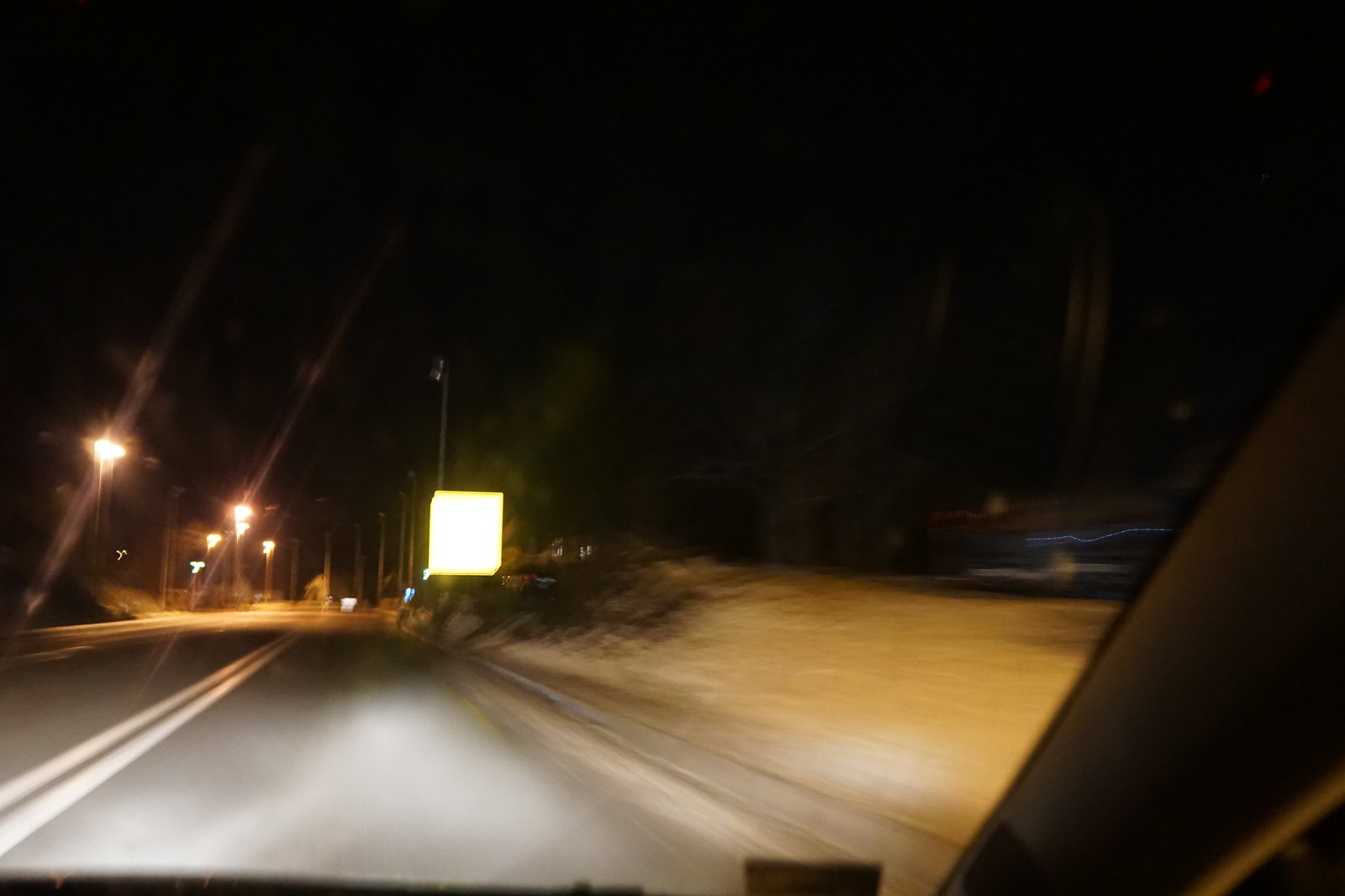The image captures a nocturnal scene through the windshield of a moving vehicle, emphasizing the pitch-black sky indicative of night. The vehicle's headlights cast a clear view of the street ahead, while the camera angle reveals the direction of travel. On both sides of the road, tall street lights cast a noticeable glare across the dark sky, adding a sense of depth and illumination to the scene. The right side of the image contains a faintly visible grassy area, accompanied by an indistinct, blurry patch intersected by a blue line, suggesting movement and creating a dynamic contrast against the otherwise sharp elements in the frame. The overall composition conveys the quiet solitude of nighttime travel with an ambient, somewhat ethereal quality.